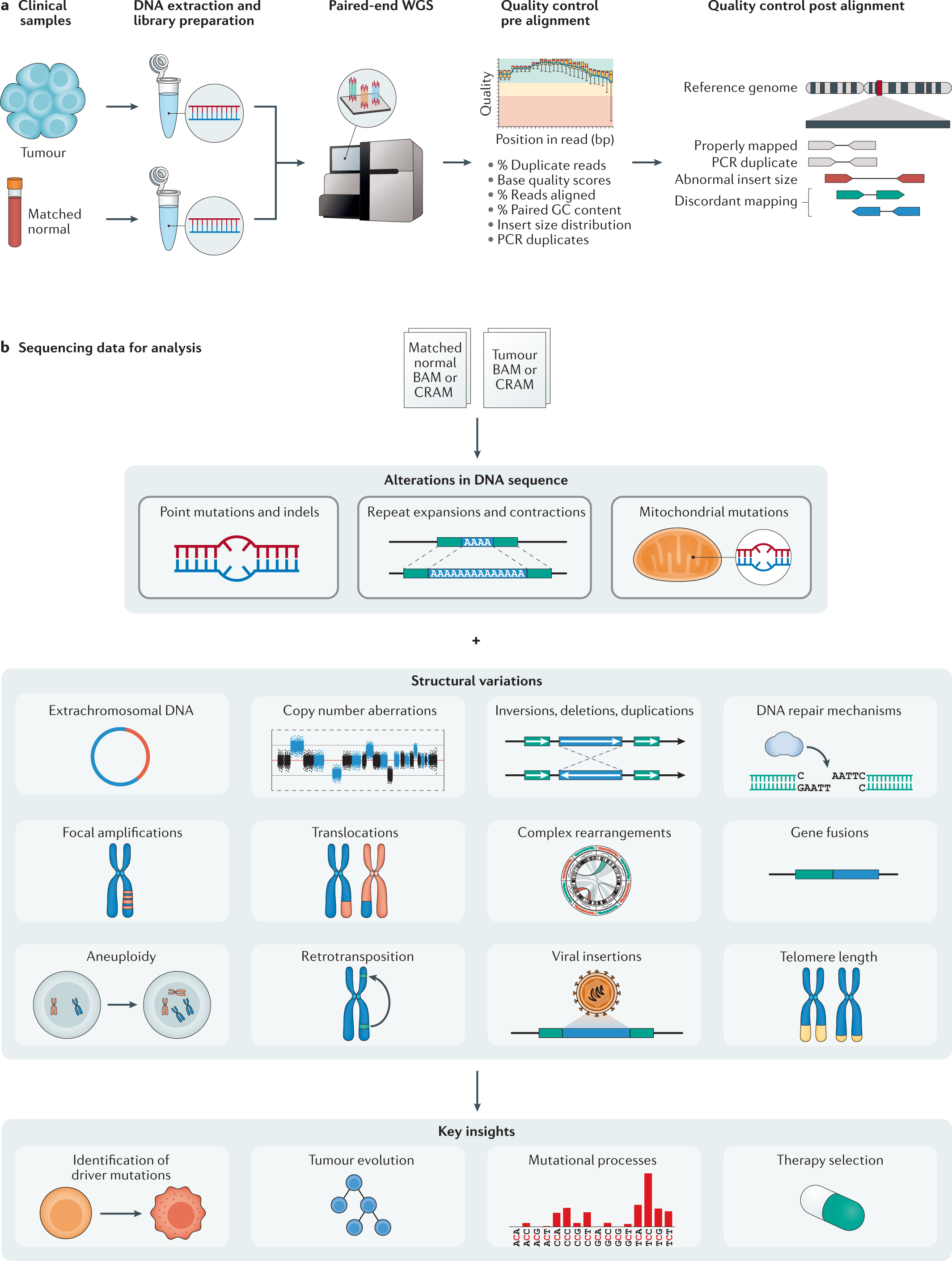The image depicts a highly detailed and colorful instructional poster or manual related to biological processes, specifically focusing on tumor genetics. Dominated by a baby blue background, the poster is adorned with an array of colors including yellow, red, teal, and black text primarily. At the top, the poster is titled "The Clinical Sample," accompanied by a hand-drawn illustration of a blue tumor. Following this, the poster outlines several stages of DNA analysis, beginning with the clinical sample, moving through DNA extraction and library preparation. Illustrated with various diagrams and labeled sections, the poster details processes such as paired end whole-genome sequencing (WGS), quality control pre- and post-alignment, tumor and normal sample comparison, and DNA sequence alterations. Noteworthy sections include structural variations with twelve illustrative images, and key insights at the bottom. The visual journey also touches on complex genomic phenomena like copy number aberrations, inversions, and mitochondrial mutations.